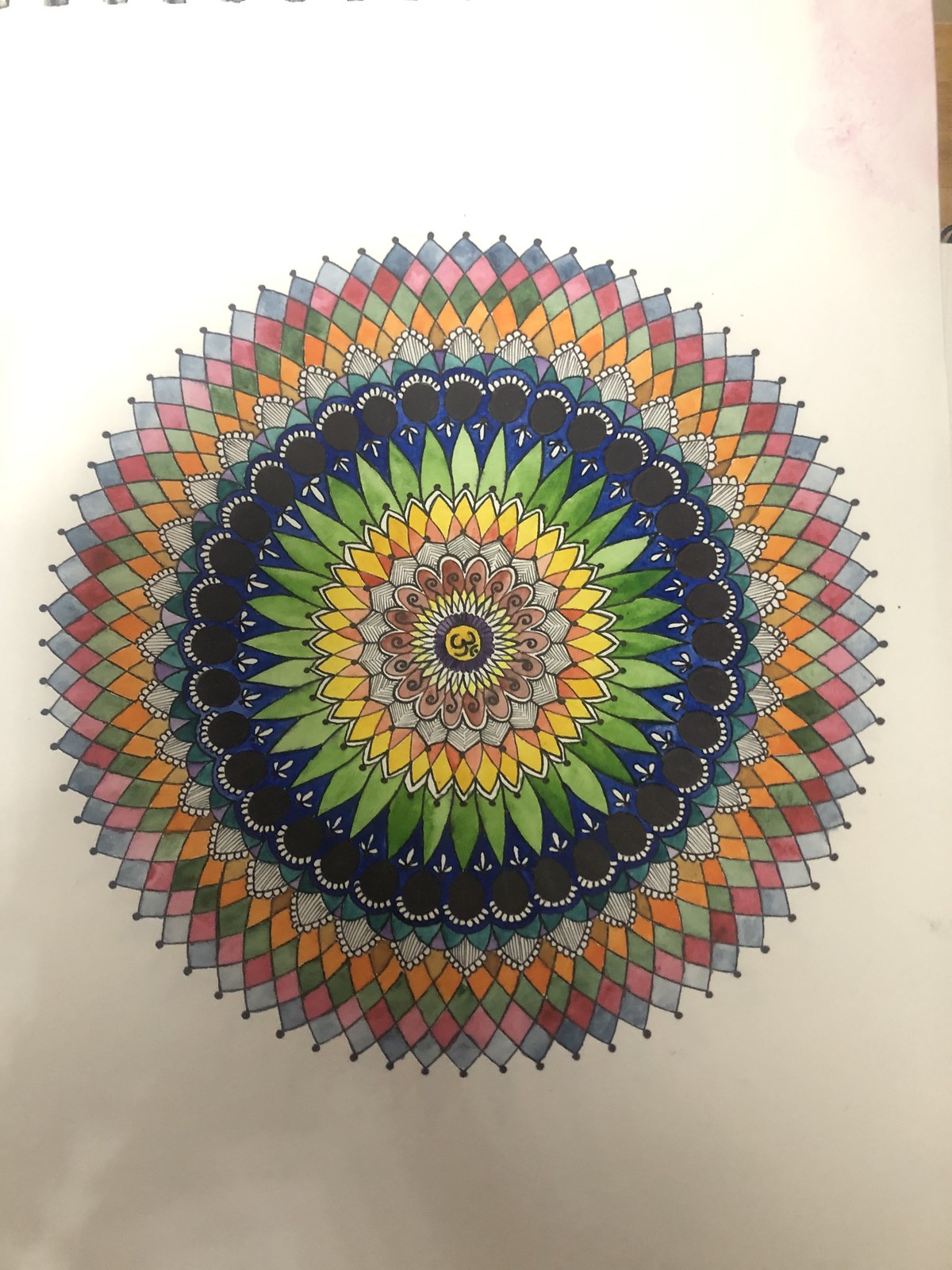This image is a photograph of a detailed color illustration of a symmetrical mandala, drawn on a plain white piece of paper that shows some shadowing and creasing. In the upper left-hand corner, metal bindings of the notebook are visible, while the upper right-hand corner exposes a medium brown wooden table with some pink smudging on the page. At the center of the mandala, there is a floral-like design that resembles a sunflower, with intricate layers radiating outward. The initial central pattern, colored in shades of brown, gold, and green, is followed by a delicate black and blue lace-like motif. Beyond this, layers include black circles with white petals, and a larger petal pattern marked by black and white stripes, ending in small black circles at the tips. The petals are vividly colored in blue, pink, green, and orange. The outermost part of the mandala features a repeating diamond pattern in alternating colors of gold, green, pink, and blue, adorned with dots all along the perimeter. No text, people, animals, or natural elements like plants or trees appear in this vertically oriented image.